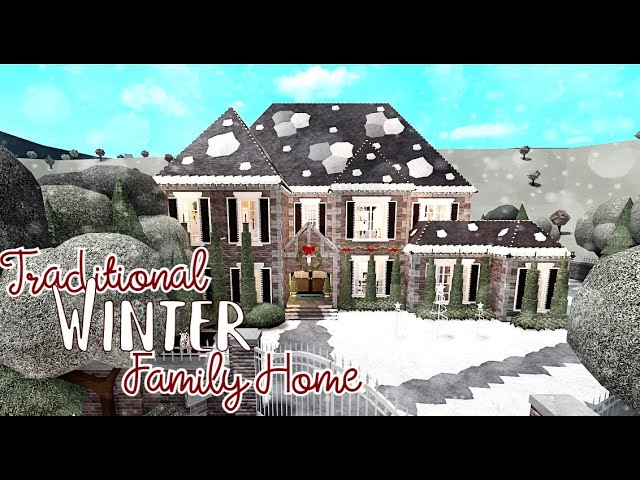The YouTube thumbnail image showcases a traditional winter family home, appearing pixelated like a house built in Sims 2. The illustration, possibly hand-drawn or computer-generated, features a two-story American-style house with text that reads "traditional winter family home." The backdrop includes a bright blue sky, creating a strong contrast. The house, situated within a gated wall, has a front garden with a white path, likely indicating snow. Patches of snow adorn the roof, and trimmed hedges surround the first floor, enhancing the impression of an expensive home ideal for a winter vacation.